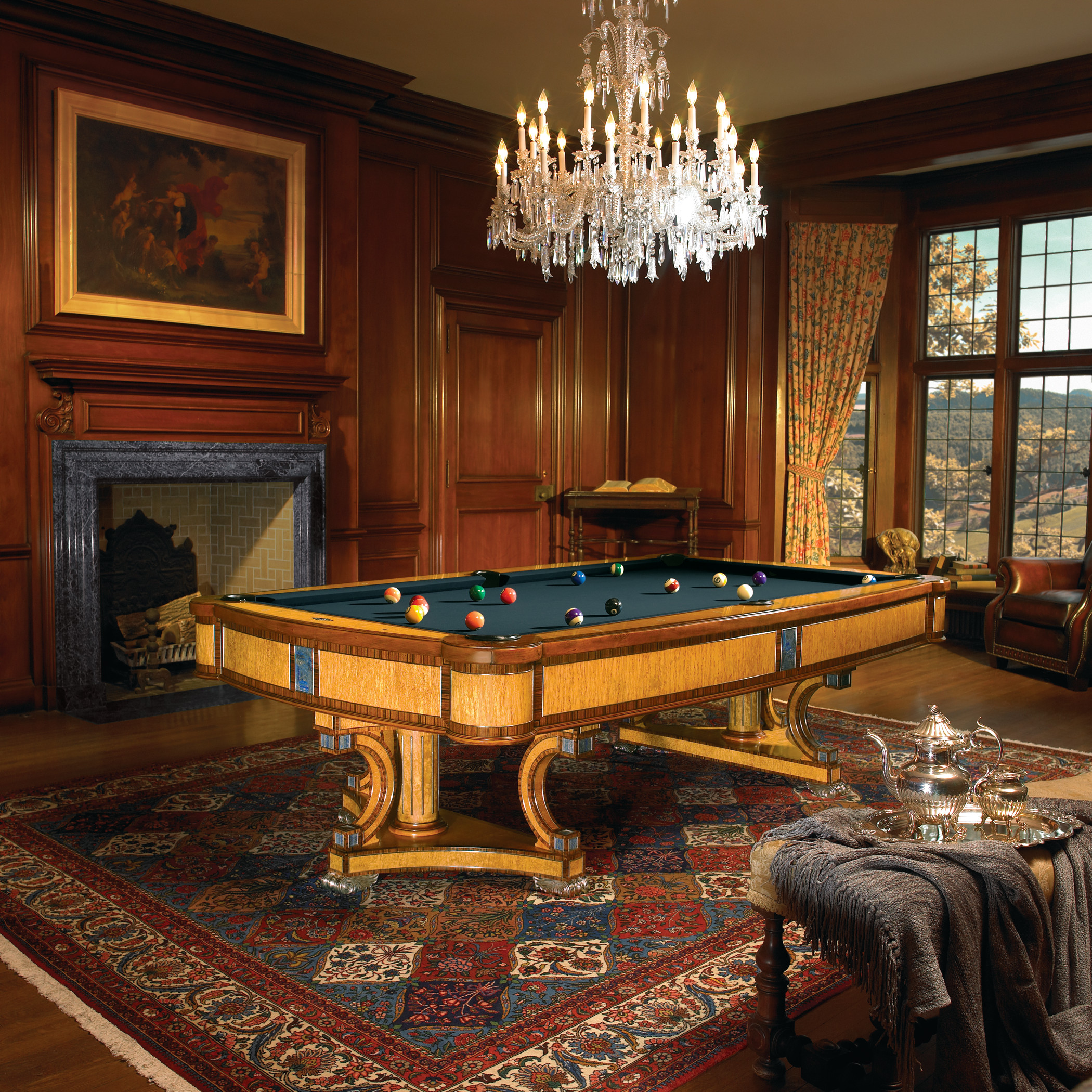In this digital photograph, we see an inviting study room with predominantly wooden walls and a rustic charm. Central to the room is a detailed, green-felt pool table laden with billiard balls. Hanging above the pool table is an elegant white chandelier featuring candle-shaped electronic lights. To the upper left, there is a painting portraying several individuals, adding a touch of historical ambiance. 

Through grid-style windows, the tranquil beauty of a mountain range and surrounding trees can be admired. The room also boasts a fireplace, its backsplash adorned with distinctive yellow square tiles, providing warmth and a cozy atmosphere. In front of the fireplace, we find a patterned rectangular carpet with rich hues of red, blue, and white, reminiscent of 17th-century designs.

Completing the setting, a leather chair and a stool can be found; the latter holds a silver tea set, including a teapot and pitcher. A metal tray and gray blankets on the bottom right add further comfort and functionality to this well-appointed space. The colors within the room harmonize in tones of brown and light brown, accented by pops of green, red, blue, and white, creating a cohesive and inviting environment.